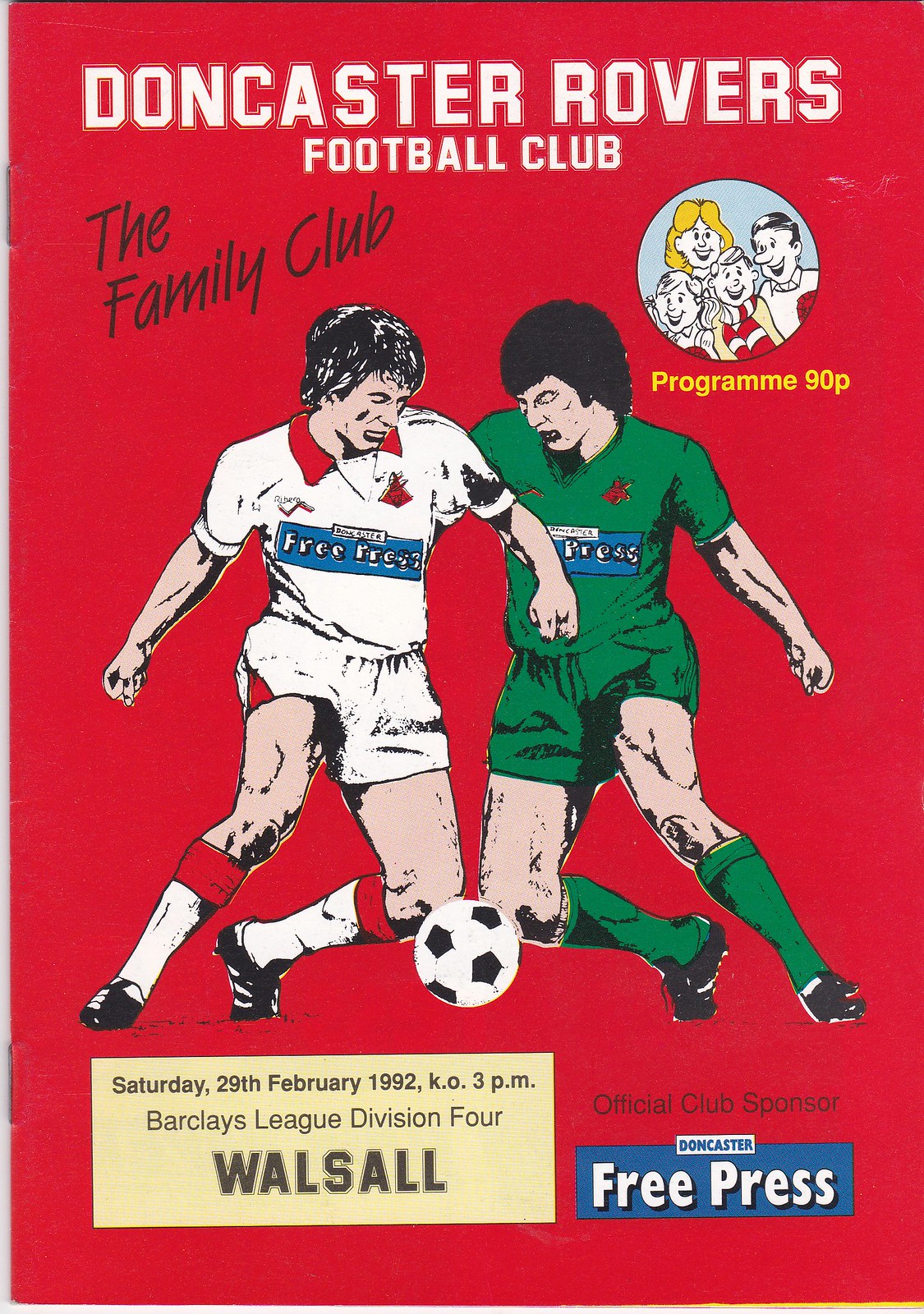The image is of a soccer program cover with a vivid red background. At the top in large white letters, it reads "Doncaster Rovers," followed by "Football Club" in smaller white letters directly below. On the lower left in black angled letters, it says "The Family Club," and to the right of this, there's a circular illustration of a cartoonish family—mother, father, daughter, and son—all smiling. Below this illustration, in smaller yellow letters, it says "Program 90P."

Prominently featured in the center are two illustrated soccer players vying for a single ball. The player on the left is dressed in an all-white outfit with black cleats, whereas the player on the right wears an all-green outfit. The soccer ball is positioned between them near their knees.

At the bottom of the image, there's a light beige rectangular area with black letters detailing the event: "Saturday 29th February 1992, KO 3 p.m." followed by "Barclays League, Division IV, Walsall." To the right of this, also in black letters, it reads "Official Club Sponsor." Directly beneath that, on a blue background, white letters spell out "Free Press." Between the "Official Club Sponsor" text and "Free Press," there's a section that says "Doncaster" in black.